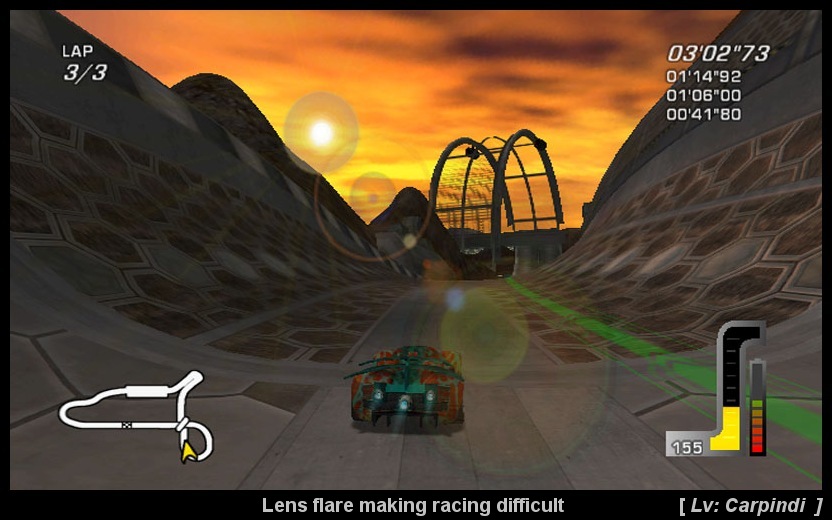The screen capture depicts a scene from a vintage racing video game set on an alpine-themed racecourse. The track features a series of sharp turns and straight stretches. The player's perspective is from behind a futuristic car equipped with triple exhausts. The car is approaching a creatively designed over-arching bridge. The distant amber-colored sun casts an eerie glow over the landscape, enhancing the game's otherworldly atmosphere. The road is bordered by embankments on both sides, which have a reptilian or space-like design, reinforcing the alien planet setting.

In the upper right corner, metrics display reads "0302" and "73," likely representing the car's current position. The upper left corner indicates that the player is on the third lap of three. A mini-map in the lower left corner shows the player's position on the racecourse, and a speed indicator on the right reads "155," accompanied by a vertical bar graph. A lens flare effect at the bottom adds to the immersive but challenging visuals. The text "LV...carpindi," possibly denotes the player's name or a specific game mode. This detailed depiction captures the essence of a vintage yet futuristic racing video game.